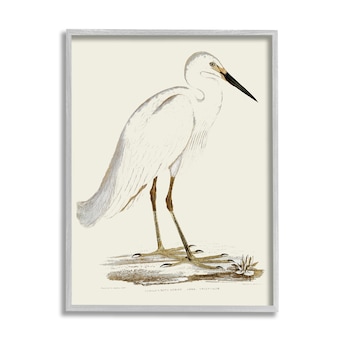This image depicts a delicately painted heron, predominantly white, with its form defined by subtle gray outlines. The heron's long beak is strikingly black, edged with touches of yellow near its eye, which itself is rendered in a lighter, less prominent tone. The bird's legs transition from a yellow ochre to a paler yellow towards its feet, ending in painted black talons standing on what appears to be a small, brown sliver of land. This land, lightly detailed, suggests a marsh-like setting with hints of flora. The entire scene is set against a stark white background, enhancing the ethereal and almost elusive outline of the heron, and is framed by a thin white frame casting a slight shadow, adding depth to the composition.